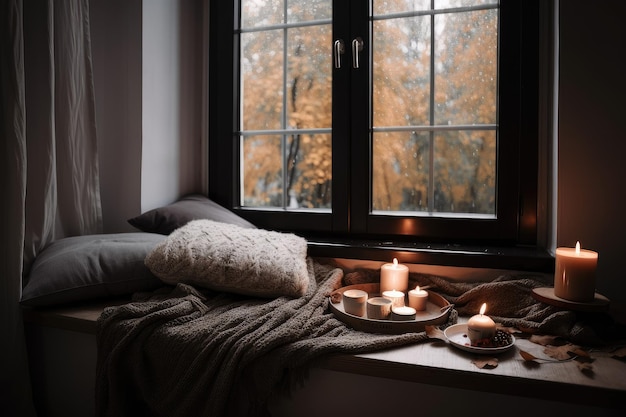A hyper-realistic rendering of a cozy bedroom window nook reveals a scene bathed in the warm glow of candlelight, perfectly setting the mood for a serene autumn day. The dark-paneled double window, which opens outwards with two small handles at the center, frames a view of orange autumn leaves on wet, dark-trunked trees, hinting at a gentle rain outside. The windowsill, easily spacious enough to sit or lie on, is invitingly adorned with a fuzzy gray blanket and three plush pillows—two dark and one white. Scattered on the blanket are autumn leaves, enhancing the seasonal ambiance. Three round dishes, including a larger platter holding six candles of varying sizes and two smaller trays each with one lit candle, add a comforting glow to the nook. Altogether, eight candles illuminate the windowsill, creating a cozy, tranquil retreat from the darkened interior of the bedroom.